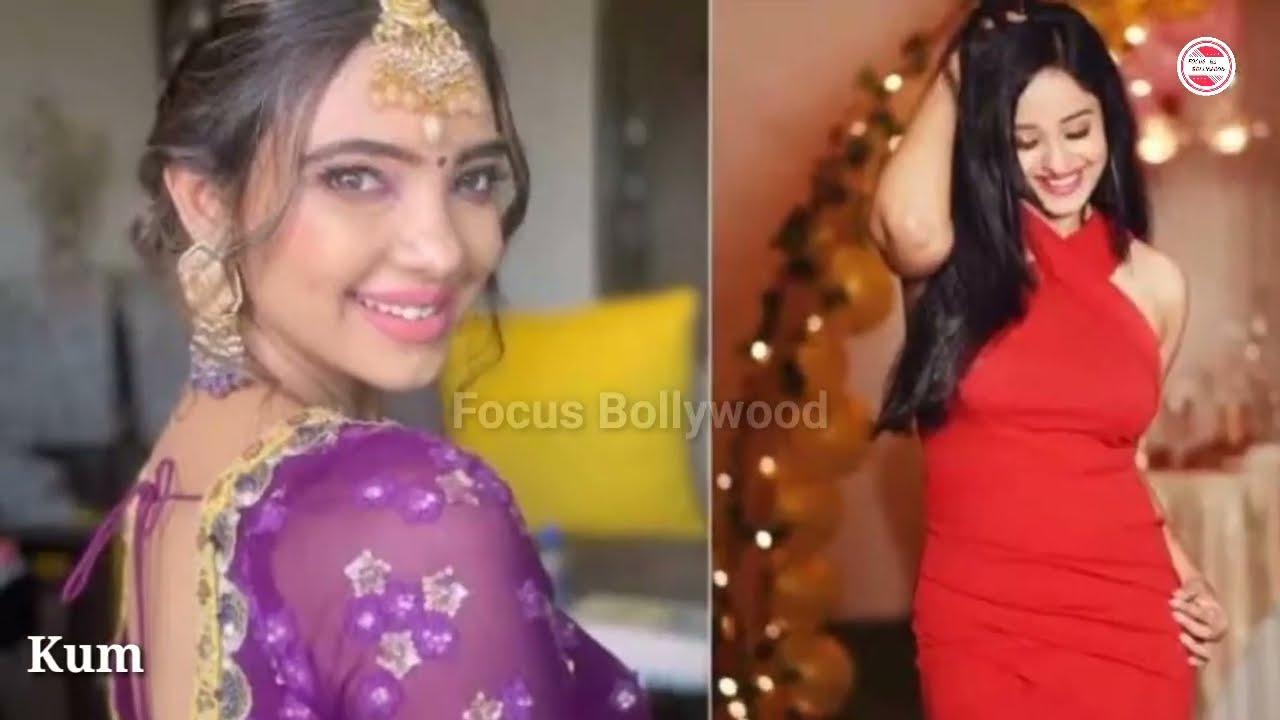This image features two photographs side by side, potentially of the same young woman. The word "FOCUS BOLLYWOOD" is prominently displayed in grayish lettering across the center, intersecting both images, suggesting a theme related to Bollywood.

In the left photograph, the young lady is seen looking back over her right shoulder at the viewer. She has dark brown hair pulled back with loose wisps framing her face, parted down the center. A large gold and white pearl amulet adorns her forehead, complemented by a black dot between her eyebrows. She wears a sheer purple top tied at the open back and a large gold earring is visible in the lower part of the image. Her happy smile adds to the charm. The background includes a yellow pillow and white walls. In white print in the bottom corner, the letters "KUM COME" are noticeable.

In the right photograph, the young lady, possibly the same, appears with natural makeup and no jewelry. Her dark brown hair is straight and loose, as she tilts her head downward with eyes closed and mouth open in a serene smile. One arm is raised behind her head, the other rests on her hip. She is dressed in a form-fitting red dress, and behind her is a gold-colored element, possibly balloons. The background includes various decorative objects like lights, flowers, and a vase. A red, white, and black symbol appears in the top right corner, though the text on it is indecipherable.

Overall, the juxtaposition of the two images with vibrant colors and intricate details - including gold, purple, red, and white tones - adds a rich, Bollywood-styled glamour to the composition.